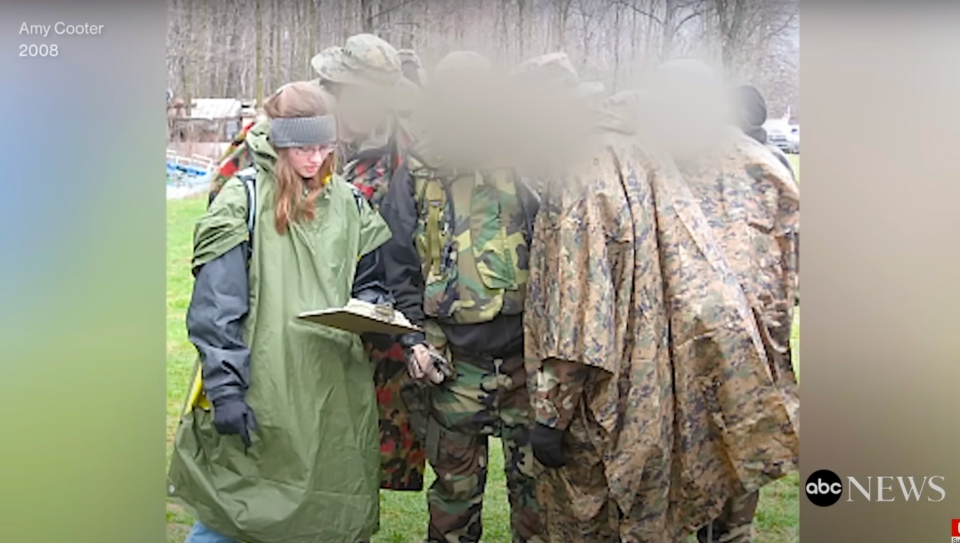The image is a horizontally oriented screenshot from a 2008 ABC newscast, as indicated by the white text "Amy Cooter, 2008" at the top left and the ABC News logo at the bottom right. The scene depicts a group of people standing on green grass with a backdrop of mostly bare trees, suggesting a winter setting. The edges of the image are blurred with narrow gray strips on each side. In the foreground, a young woman with blonde hair, glasses, and a headband is prominently visible. She is wearing a green raincoat with black sleeves and gloves, and she's holding a clipboard with papers attached to it. Surrounding her are three individuals, presumably men, dressed mostly in camouflage or rain gear. Their faces are obscured by gray ovals, making them indistinct. Additional figures are faintly visible in the background but remain blurry and indistinct, focusing the attention on the young woman and her clipboard.